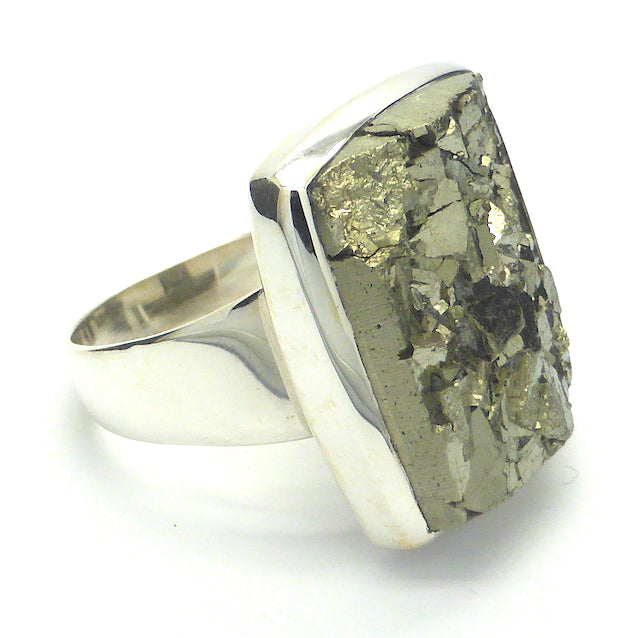This photograph captures a floating, three-dimensional silver ring with a thick band set against a pristine white background. Positioned on its side, the ring's centerpiece commands attention—a stunning, large square stone that dominates the top of the ring. This natural stone or geode features a captivating mix of grayish-greenish-gold hues, reminiscent of fool's gold, with a jagged, rough, and unpolished texture. The stone is nestled within a silver border that transitions into a bronze-gold base with a swirling pattern of white and gray. Subtle shadows beneath the ring and dark reflections on the metal band add depth to the composition, emphasizing the ring's intricate details and robust design.